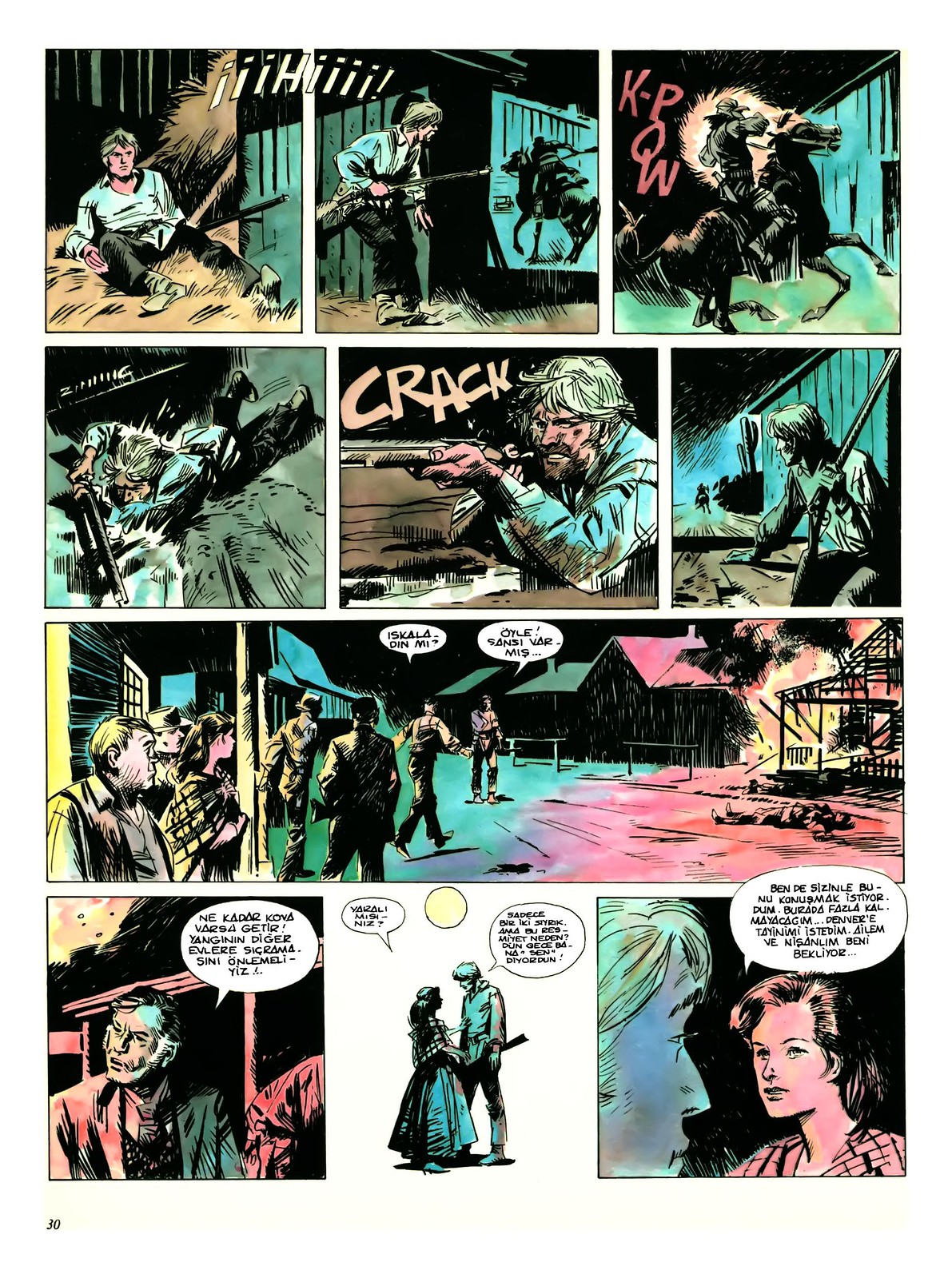This is a classic comic strip set on a single page segmented into several panels, specifically laid out in a structured grid. The page, marked as number 30 in the bottom left-hand corner, unfolds a dramatic sequence in an Old Western setting with a consistent color palette of blues, reds, and tans, giving it a distinctive sketchy feel.

At the top of the page, the first three panels depict a blonde, white man in a long-sleeve white shirt and gray pants laying in hay inside a barn. The following set of three panels transitions into a tense encounter—this man is shown wielding a rifle, aiming at another figure on a black horse. The narrative progresses with sound effects like "Hi," "Kapow," and "Crack" illustrating the gunfire, as the mounted figure appears to be shot.

Spanning the entire width of the page beneath these panels is a long, single panel showing two people conversing. Text bubbles in a non-English language suggest dialogue, presumably about the escalating confrontation, set against what appears to be a burning farmhouse.

Below this expansive panel, three more segments continue the story, showcasing the man with the gun hiding beside a building as bystanders approach, furthering the tense atmosphere with more dialogue also encompassed in non-English text bubbles. This meticulously detailed comic page vividly captures a moment of high suspense with its dynamic imagery and expressive colors.